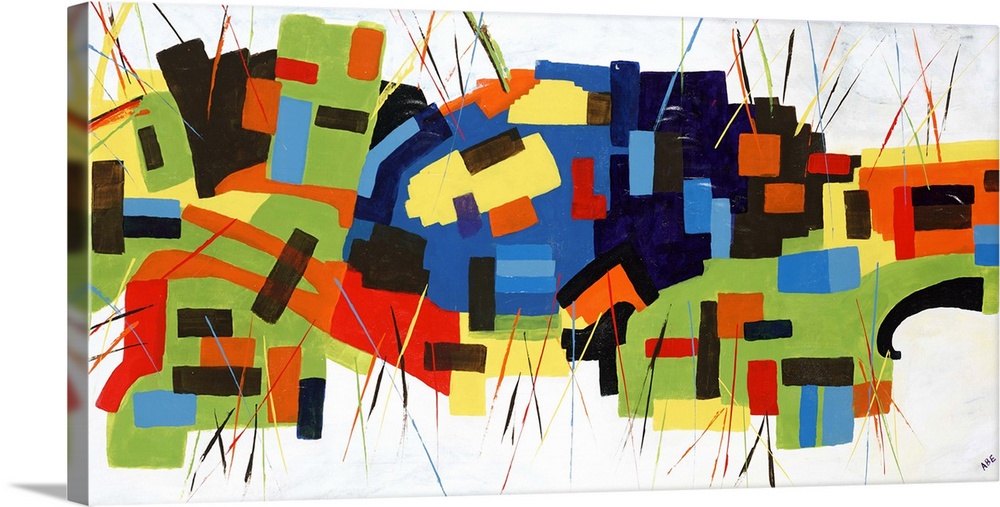The artwork depicted is a vibrant and abstract piece set on a rectangular, all-white canvas, oriented with its longer side as the base, approximately two feet wide and one foot tall. The painting uses a plethora of bold primary colors like red, orange, royal blue, light blue, green, yellow, and black, along with additional shades such as navy blue, light blue, purple, pink, beige, tan, and brown. 

The composition of the image appears chaotic but visually stimulating, featuring a dense collection of geometric shapes including squares, rectangles, and 'L' shapes that intersect and overlap without any discernible pattern. Vibrant lines, some reminiscent of toothpicks or pen strokes, extend out to the edges and corners of the canvas, contributing to the dynamic appearance. The center of the painting is notably dominated by black and bright blue, with a concentration of green towards the bottom right and left sections.

Adding to its 3D effect, the image is photographed from an angle that reveals the side strip of the canvas, which is also painted, suggesting continuity of the abstract design even on the sides. At the bottom corner of the canvas, there is a text written diagonally in blue or purple, spelling "A-B-E." Shadows cast on an all-white background from the artwork emphasize its three-dimensionality. 

The bottom right part of the canvas seems to depict an abstract representation of a house with a black-bordered red structure, orange walls, black windows, green grass in front, a black curb, and a blue corner. The vivid portrayal is enriched with sporadic blotches and streaks of colors, invoking an intense, dynamic aesthetic.